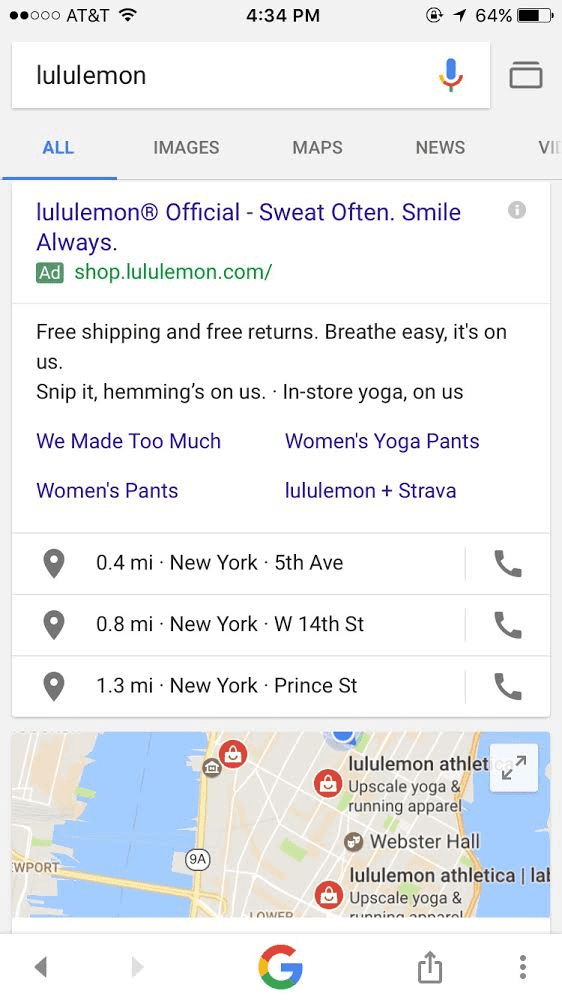This screenshot captures a mobile device's screen displaying the Google app in use. At the very top of the screen, the status bar shows five notification dots, with two highlighted in black, indicating active notifications. The status bar also reveals the carrier AT&T, a Wi-Fi icon, the current time (4:34 PM), an orientation lock icon, a location active icon, and a battery icon displaying 64% charge.

Below the status bar, the Google search interface is visible. The search query entered is "lululemon." To the right of the search bar, there is a microphone icon for voice searches. 

Just beneath the search bar, navigation tabs for different types of results are displayed: All, Images, Maps, and News, with the word "video" partially visible but cut off. The "All" tab is currently active.

The first result is an advertisement for Lululemon, tagged with the slogan "sweat often, smile always," and links to the URL shop.lululemon.com. Beneath this ad, additional search results are partially visible, including an embedded map at the bottom of the screen. This map section displays various store locations, complete with addresses, distances, and clickable phone icons for contact information.